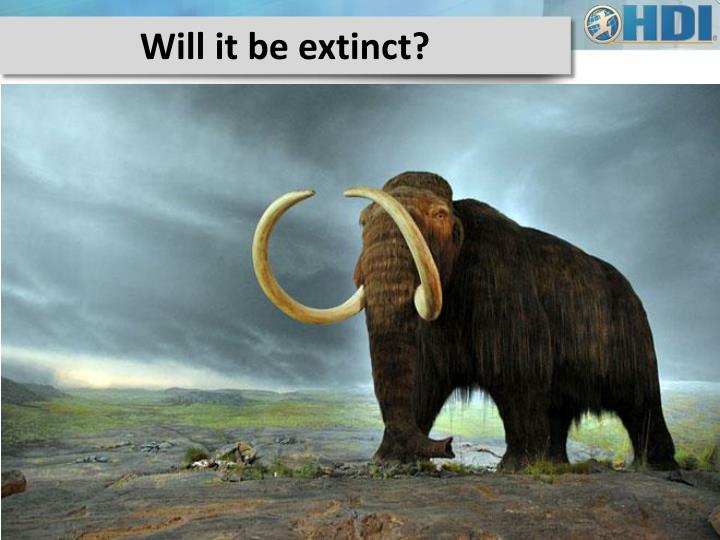This image, which resembles a lifelike drawing or slightly blurred photo, features a woolly mammoth standing on a rocky, arid landscape. The mammoth, with its large, imposing tusks and shaggy, blackish-brown fur, is positioned facing left but looking slightly forward. The backdrop comprises a cloudy, stormy sky that extends down to the horizon, leaving only a small clearer section in the lower left. Above the mammoth, a white bar contains the text "Will it be extinct?" in black font, with the "W" capitalized. In the top right corner, the emblem of a silver figure with outstretched arms in front of a globe is visible, next to the blue letters "HDI." Sparse shrubs or grasses are hinted at in the distance, enhancing the arid yet slightly green terrain.